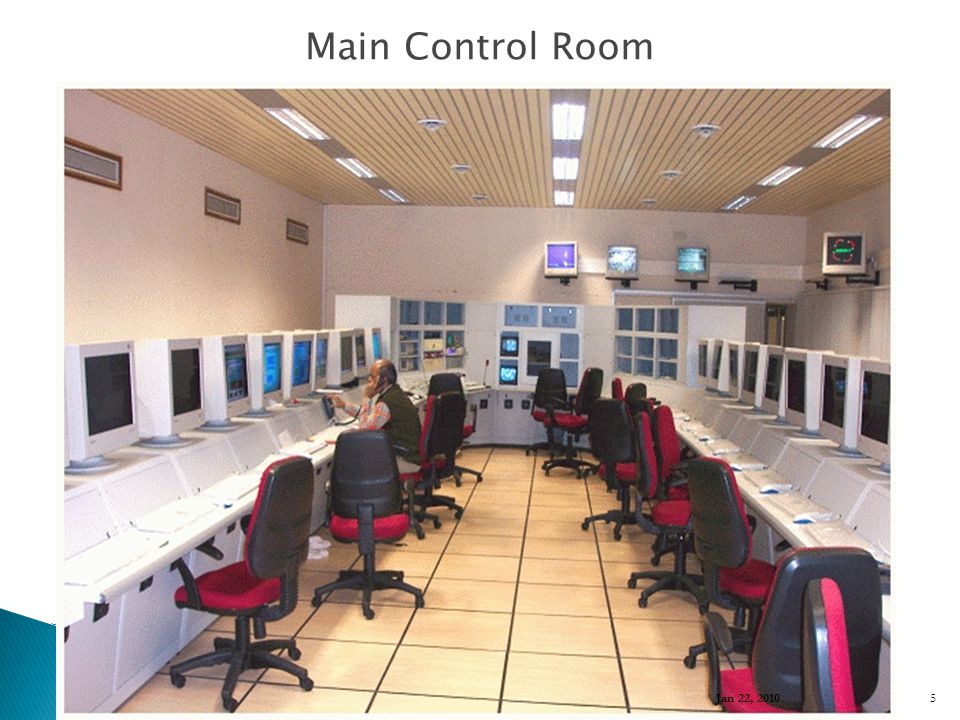The image depicts a main control room, prominently labeled at the top with the text "main control room" in black. The room features a beige tile floor with dark grout and is filled with around 20 or more large, older model computers arranged in a U-pattern and in rows along the walls. These computers have thick white screens reminiscent of technology from the 1990s or early 2000s. There are approximately 16 red office chairs with rolling black legs and black structural elements. The room's ceiling is lined with three rows of fluorescent lights and features a wooden board design with additional built-in lights.

On the left side of the image, there are three rectangular windows, while the right side and center contain several monitors, some of which are likely used for security or other types of monitoring. Notably, a more advanced control station with multiple smaller screens is positioned at the back of the room. Among the computers, about 6 to 8 monitors are turned on, while the rest remain off. One man is visible, situated on the left side of the image, seated at a computer and talking on the phone. Embedded into the bottom corners of the image are a date, January 22, 2010, and a small fine print label, number five. This detailed control room, which could belong to a power plant, a dam, or a similar facility, reflects the technology and design of an earlier era.